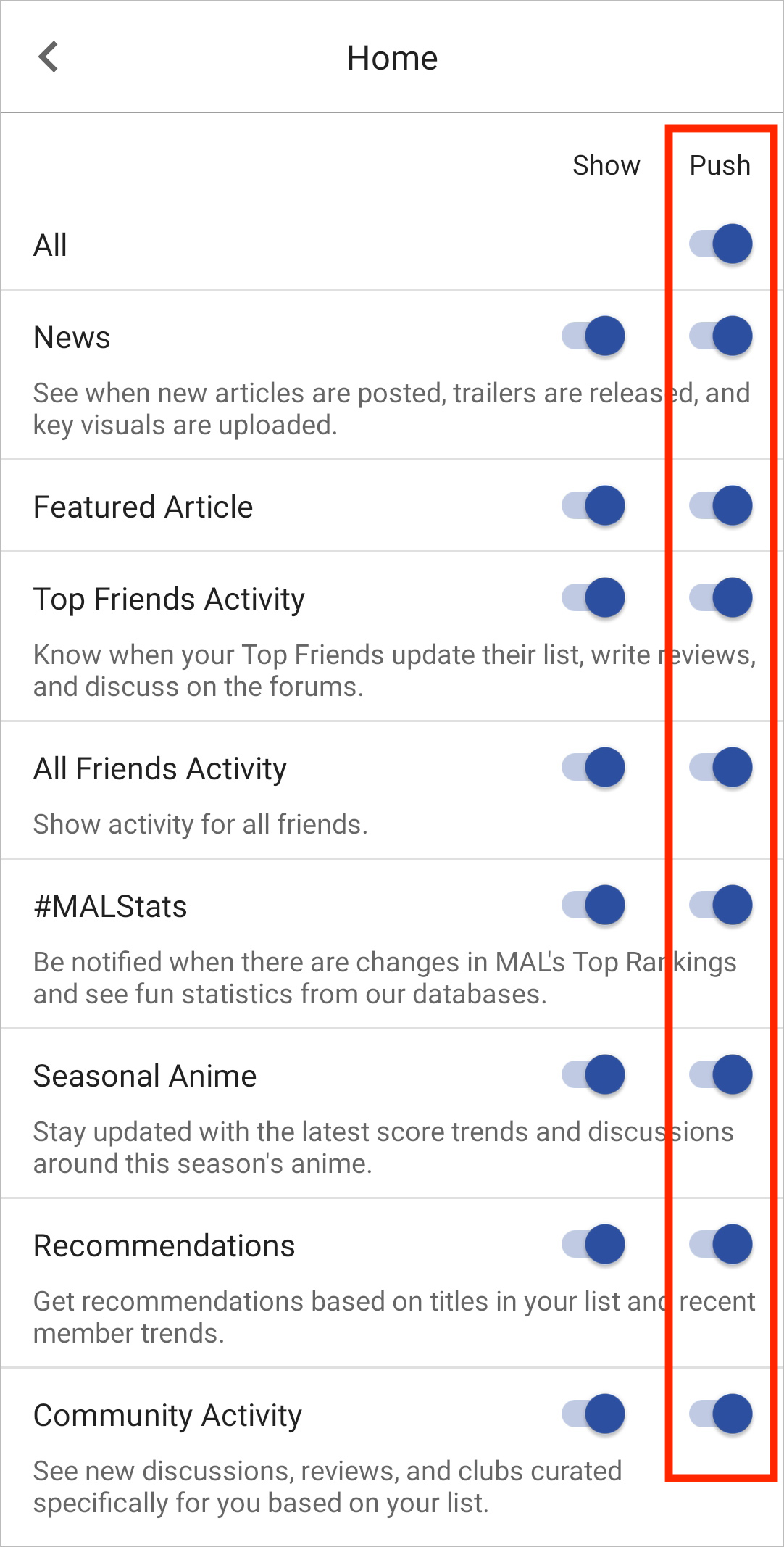The image features a user interface with a white background and black text at the top that reads "Home." On the right side, there are two sections labeled "Show" and "Push." The "Push" section is outlined with a red vertical rectangle, highlighting the various toggles within it. All toggles under both "Show" and "Push" are switched on and are displayed in blue.

Within the outlined "Push" section, the toggles correspond to various content categories:
1. **All:** Includes all content types.
2. **News:** Notifies about new articles, trailer releases, and key visual uploads.
3. **Feature Article Top Friend Activity:** Provides updates when top friends update their lists, write reviews, or discuss on forums.
4. **All Friend Activity:** Shows activity for all friends.
5. **Hashtag Trends:** Sends notifications when there are changes in top rankings and fun statistics from the database.
6. **Seasonal Anime:** Keeps users updated with the latest trends and discussions about the current season’s anime.
7. **Recommendation Guide:** Provides recommendations based on titles in the user's list and recent member trends.
8. **Community Activity:** Displays new discussions, reviews, and club activities curated specifically for the user based on their list.

The "Show" section, positioned to the left of "Push," contains the same categories but does not have the red outline.